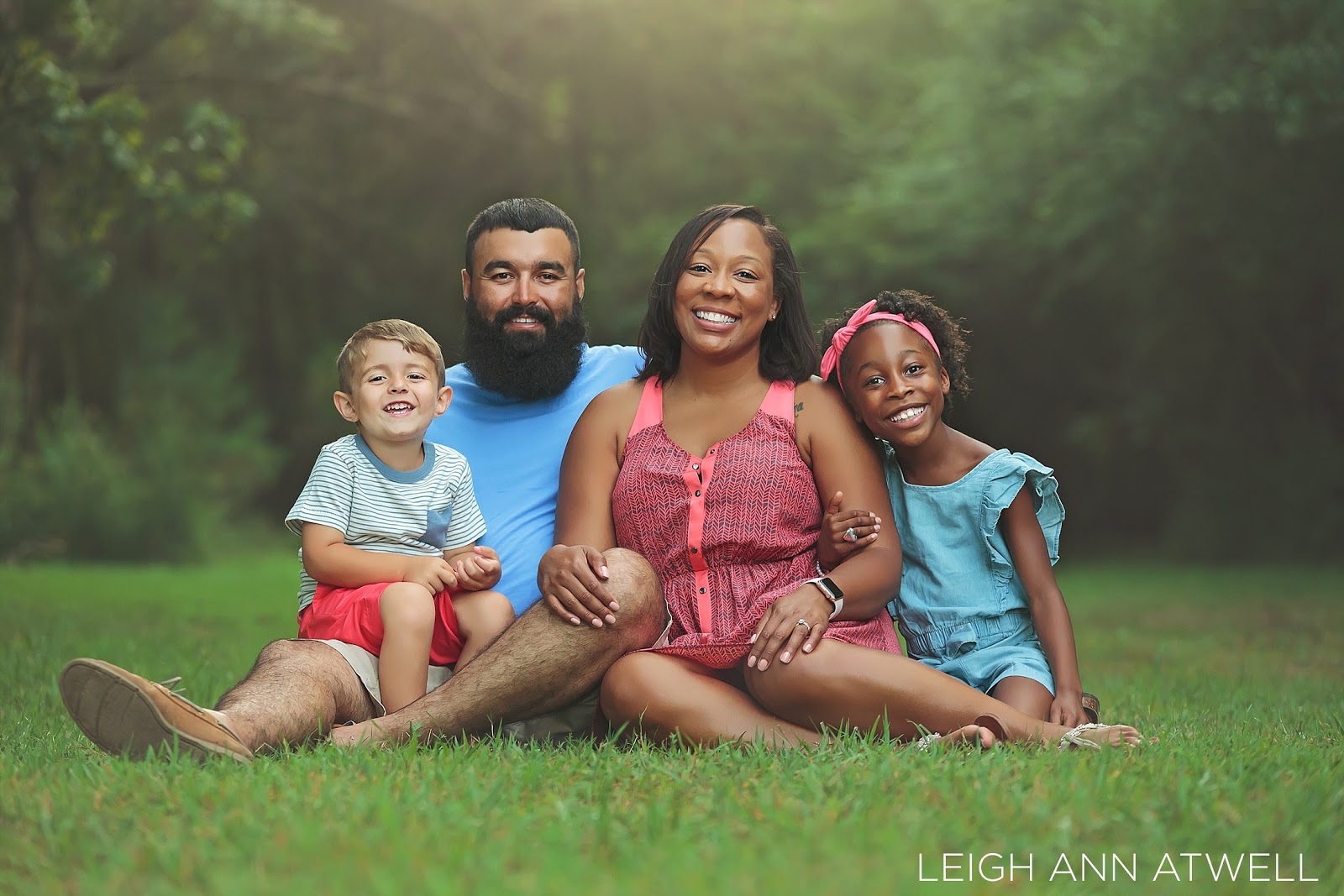The photograph is a heartwarming, professional family portrait of a mixed-race family sitting closely together on bright green grass with a blurred wooded background. The African American mother, who wears a pink outfit, has one hand gently placed on her leg and the other on her bearded partner's knee. She is adorned with an engagement ring and an Apple Watch. Her daughter, also African American, dressed in a light blue dress with frilly armholes and a pink bow in her hair, lovingly wraps her arm around her mother's. The father, a white man with a beard, is wearing a blue shirt and visible tennis shoes, and his white son, donned in red pants and a white shirt with blue stripes, sits comfortably on his lap. The photo captures them all gazing towards the camera, with "Lee Ann Atwell" signed in white lettering in the bottom right corner.